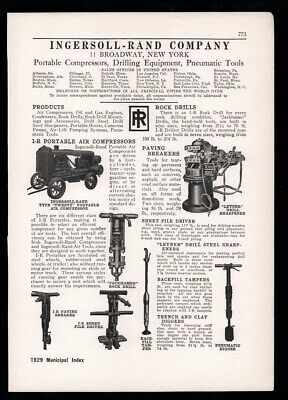This vintage newspaper advertisement from 1929 prominently features the Ingersoll Rand Company, located at 11 Broadway, New York. The ad showcases a range of their early 1900s-style industrial equipment, all depicted in detailed black-and-white images. At the top of the ad, large bold text reads “Ingersoll Rand Company,” followed by “Portable Compressors, Drilling Equipment, Pneumatic Tools.” 

The visual layout includes multiple sections labeled "Products," "Rock Drills," and "1R Portable Air Compressor," with descriptive illustrations. The "1R Portable Air Compressor" is depicted as a wheeled contraption featuring tanks and pipes. Below these, the "Paving Breakers" section illustrates a device with a black base, cables, and an unfamiliar top apparatus, alongside other pictured tools resembling various types of drills and levers. 

While much of the smaller text is difficult to read due to the paper's faded condition, the bottom left-hand corner clearly shows the date, “1929,” identifying the year of the publication and tying the advertisement to its historical context.